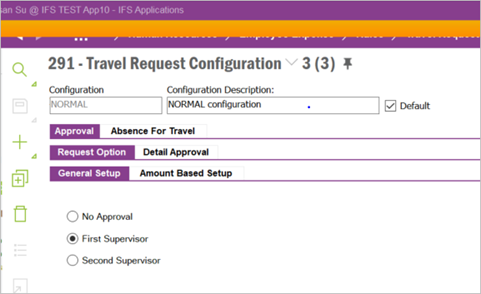### Detailed Descriptive Caption:

The web page features a distinctive purple ribbon across the top, displaying white text. At the very top, the text includes an "at" (@) symbol followed by "IFS Test App 10 - IFS Application". Below this, the white text has been hidden beneath an orange ribbon that also spans the entire width of the purple ribbon.

Just below the orange ribbon, in navy blue text, it reads "291 - Travel Request Configuration" followed by a down arrow symbol, the number "3", and another "3" enclosed in parentheses, next to a pin icon. 

Underneath, there is a section with a white box labeled "Configuration" in navy blue text. Inside this box, it states "Normal". To the right, the phrase "Configuration Description" is displayed, and inside another white box, it specifies "Normal Configuration". Adjacent to this, there is a checkbox for setting it as the default, which is currently checked.

Further down, three vertically aligned purple tabs with white text can be seen. They are labeled "Approval Request Option", "General Setup", and "Information". To the right of these tabs, information is presented within a white box bordered by purple.

 The layout is structured and color-coded to differentiate various sections and options, enhancing navigation and usability.